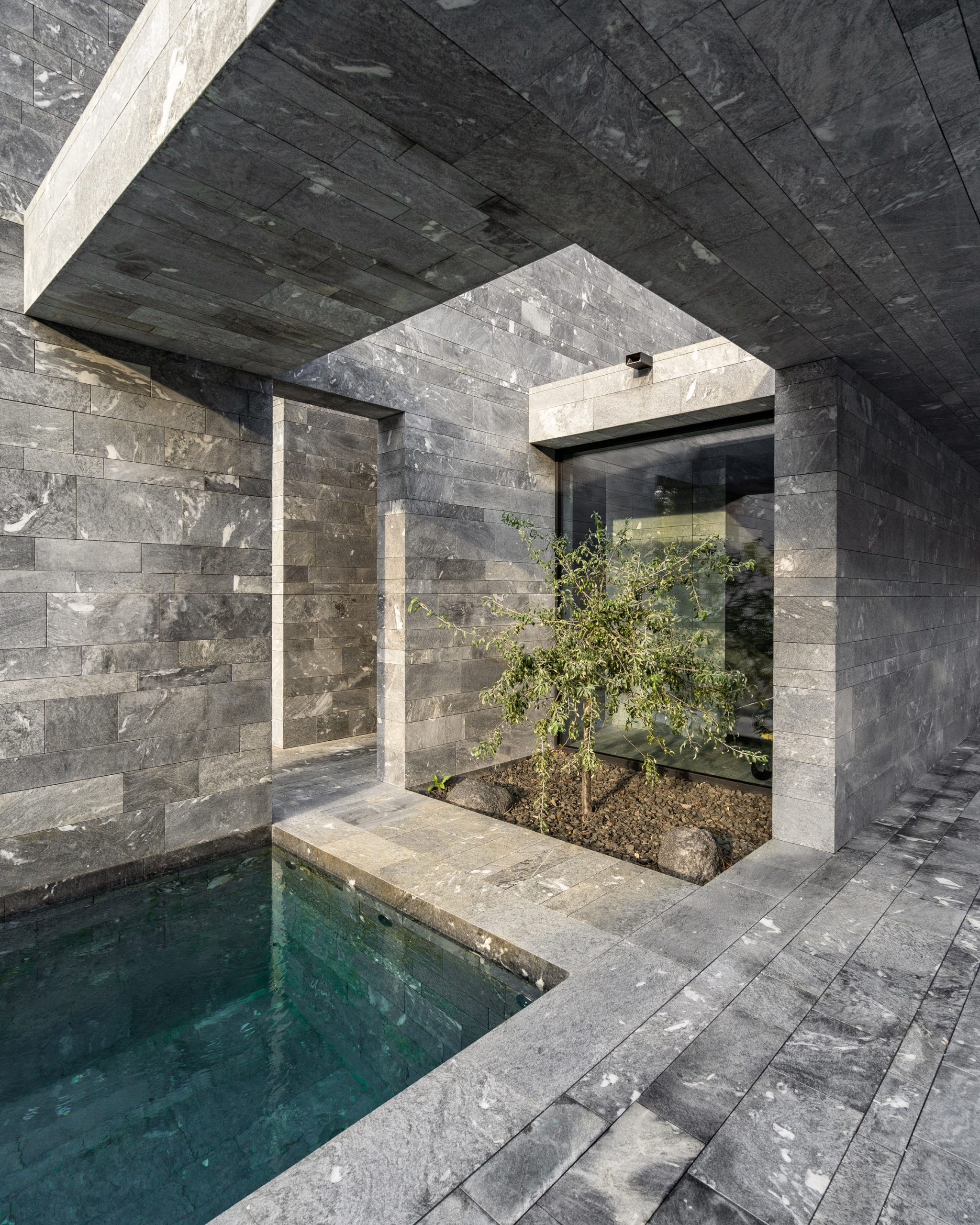The image depicts an architectural design of a modern, cement outdoor area characterized by a stark, gray color palette and straight lines. At the center is a large square window, in front of which a small tree grows from a soil bed framed with brown rocks. Adjacent to the tree is a narrow, rectangular pool filled with deep turquoise water, giving the space a reflective quality. The area surrounding the tree and pool is constructed with gray bricks or cement, giving a uniform, industrial appearance. A doorway is visible to the left of the tree, possibly leading to another part of the building, while an opening in the roof above the tree allows sunlight to penetrate the space. This section, possibly an atrium, suggests a blend of indoor and outdoor elements, emphasizing minimalistic and boxy architecture.